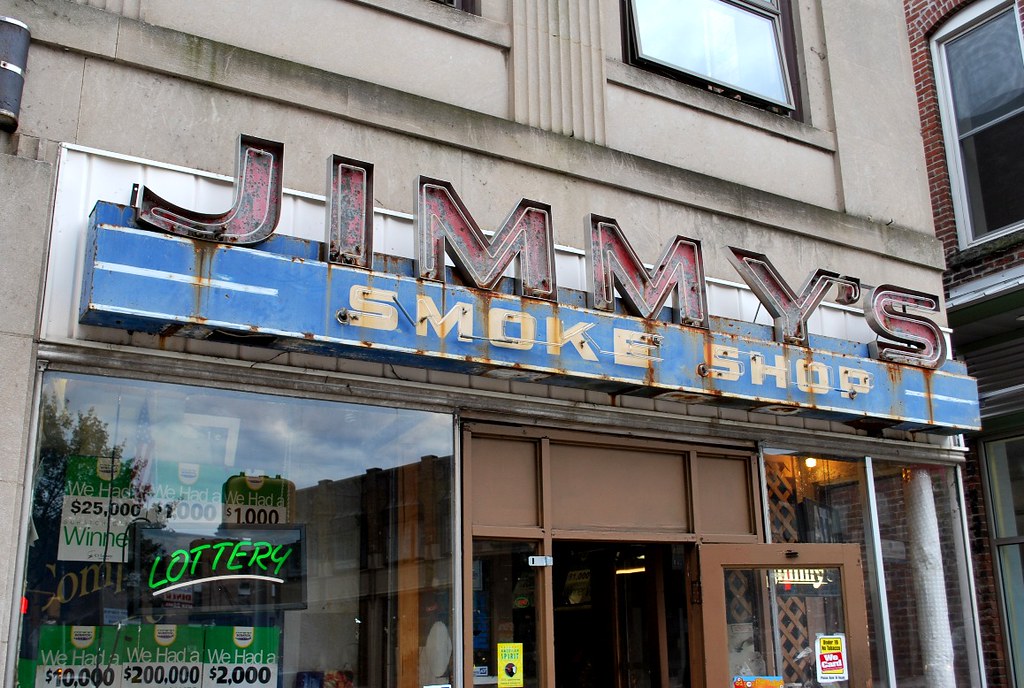The image depicts the exterior of Jimmy's Smoke Shop, situated at the base of a taller, light brown stone building. The shop's weathered and rusted sign is prominently displayed, reading "Jimmy's" in large red letters with a blue rectangular banner beneath it that states "Smoke Shop" in slightly smaller yellow letters. The building shows signs of aging, with a bit of moss suggesting prolonged exposure to rain. A neon "Lottery" sign in green letters, accented with a white underline, is visible in the window to the left. This window showcases previous lottery winners with various amounts displayed, such as $25,000. The entrance features a brown door and matching brown door frame. Overall, the image provides a detailed look at the aged yet eye-catching facade of the smoke shop, set against the backdrop of a taller building with white-framed windows.